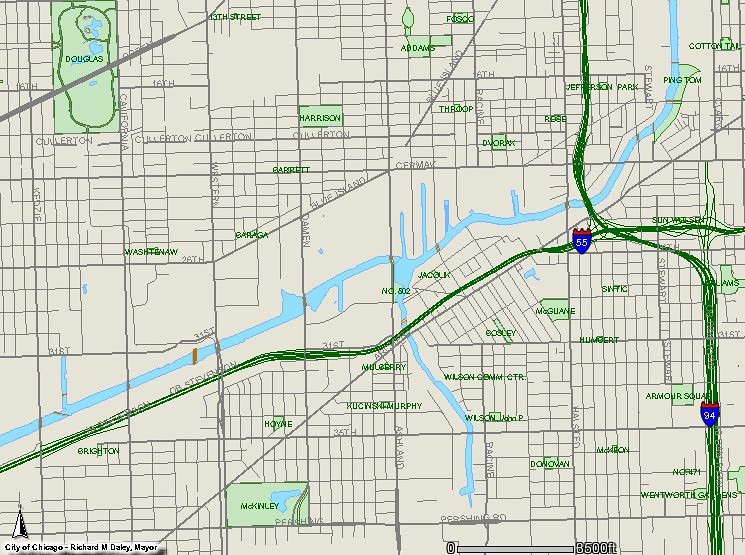The image depicts a detailed map of the city of Chicago. At the bottom, the text reads "City of Chicago - Richard J. Daley, Mayor." The map features several streets, such as 59th and 94th, highlighted in green lines. Various neighborhoods are delineated with black lines and labeled with names like "Douglas" and "Barrett." The text is somewhat shaky and unevenly spaced, with some fonts appearing blocky and closely packed. A river is shown with a thick light blue line, accompanied by brown segments indicating bridges. Additionally, a gray scale at the bottom left of the map indicates distances, ranging from 0 to 800 feet, providing a reference for map measurements.